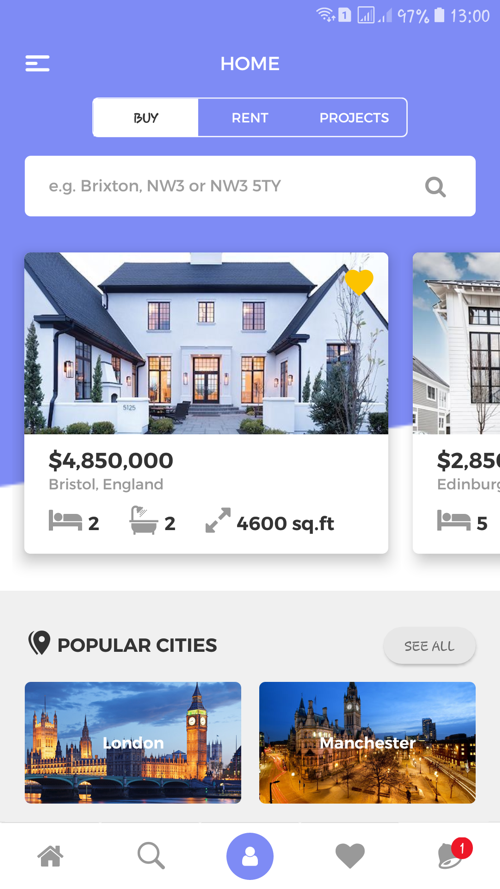The image is a detailed screenshot of a cell phone screen, easily identifiable by the symbols at the top right which include icons for Wi-Fi, calendar, cellular signal (3 out of 4 bars), battery life at 97%, and the time displayed as 13:00. The background of the screen transitions from a light blue at the top to white at the bottom.

At the very top of the screen, the navigation options are visible, with 'Home', 'Buy', 'Rent', and 'Projects' tabs, with 'Buy' highlighted with a white background. Below these tabs, there is a prominent white search bar with placeholder text suggesting possible search entries, such as "E.g., Brixton, NW3 or NW35TY."

The main content features an image of a two-story house with a courtyard or walkway, listed for sale at $4,850,000 and located in Bristol, England. The property details indicate it includes two bedrooms, two bathrooms, and spans 4,600 square feet. 

Beneath the property listing, within a light blue box, a location symbol is paired with the text 'Populous Cities' and an oval button on the right that says 'See All'. An image below this probably shows famous landmarks like a London castle with Big Ben and another tall clock tower in Manchester, both captured from an aerial view.

At the bottom of the screen, there are icons for 'Home', 'Search', 'Account', 'Favorites', and 'Notifications'. The notification icon, positioned at the bottom right, has a red circle with the number 1, indicating a new notification. The image contains no additional text.